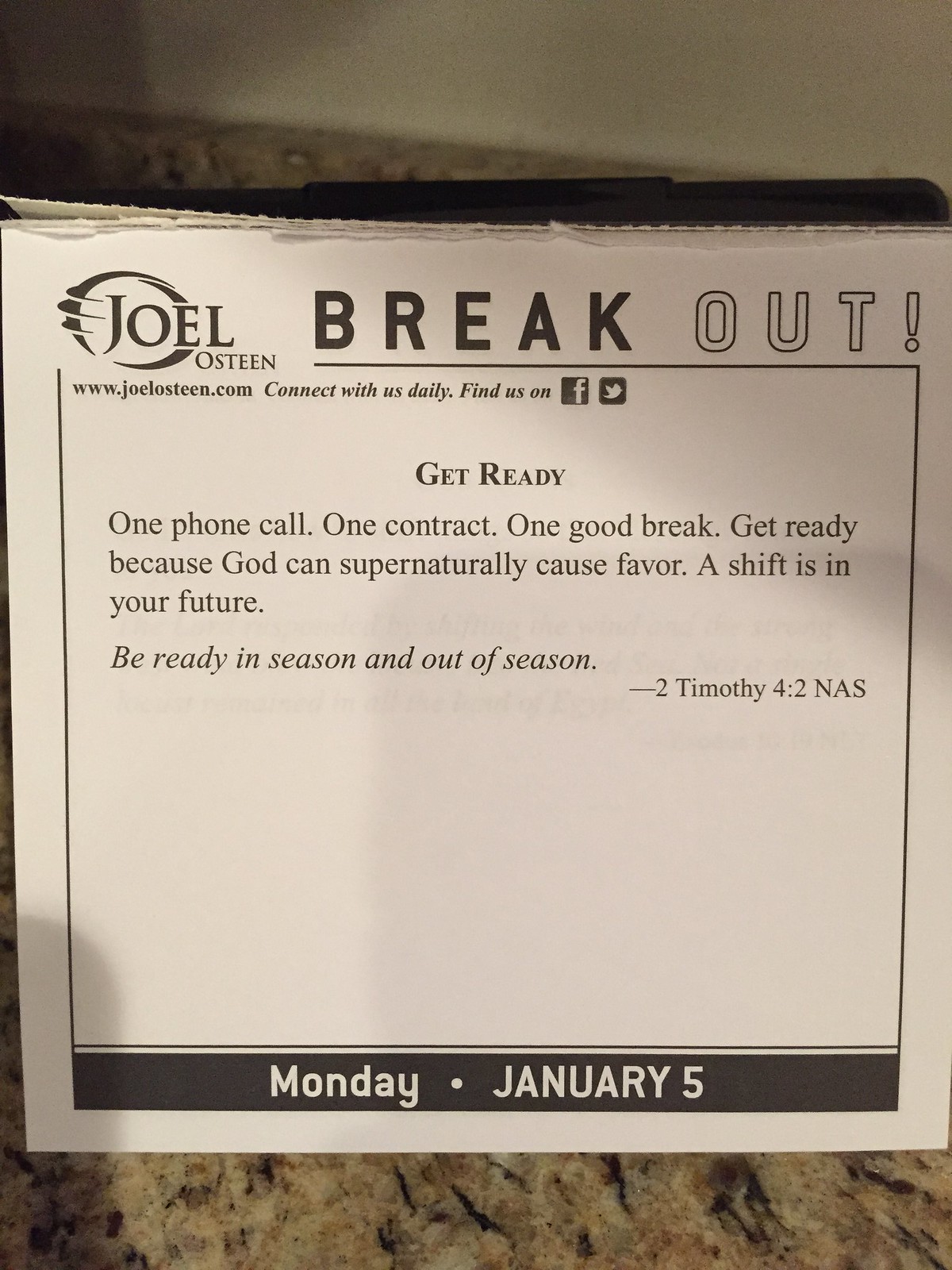The black-and-white image depicts a square, computer-printed flyer on a marble countertop, featuring Joel Osteen's logo—a stylized letter "O" with intricate markings. The title at the top reads "Breakout!" in large black letters, followed by the URL "www.joelosteen.com" and the call to action "Connect with us daily." Social media icons for Facebook and Twitter are displayed below, with the text "Find us on." The main body of the flyer contains the inspirational message: "Get ready. One phone call, one contract, one good break. Get ready because God can supernaturally cause favor. A shift is in your future. Be ready in season and out of season," followed by the biblical reference "2 Timothy 4:2 NAS." The bottom of the flyer indicates the date "Monday, January 5th," suggesting it might be a page from a tear-off calendar.